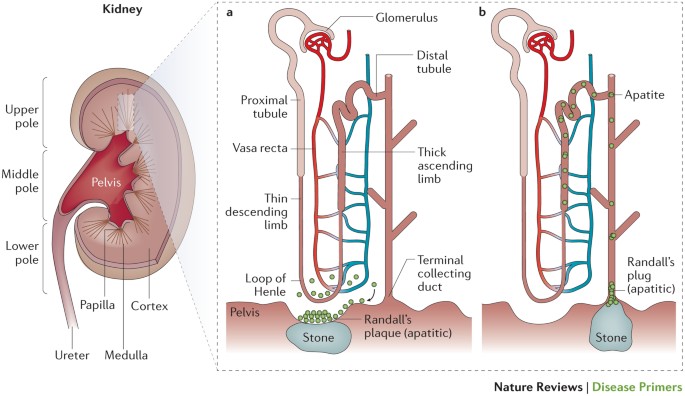The image is a detailed and contemporary poster illustrating the anatomy and pathology of kidney stones. On the upper left-hand side, there's a cross-section of a kidney, meticulously labeled with parts such as the upper pole, middle pole, lower pole, papilla, cortex, ureter, and medulla. Thin black lines connect each label to the relevant section, ensuring clarity. The kidney is shown in red and beige tones, highlighting the different anatomical structures.

Further illustrations adjacent to the kidney provide additional insights. They depict the formation and location of kidney stones, with one showing a blue kidney stone and others featuring small green dots labeled as Randall's plaque and Randall's plug. These green dots are likely indicative of the initial calcium deposits that can lead to stone formation. The use of colors like blue, green, and gray enhances the informational value, making this diagram a valuable resource for medical education, perhaps suitable for a textbook or a PowerPoint presentation. The poster provides a clear, step-by-step visualization of how kidney stones develop, labeled comprehensively to guide the viewer through the process.